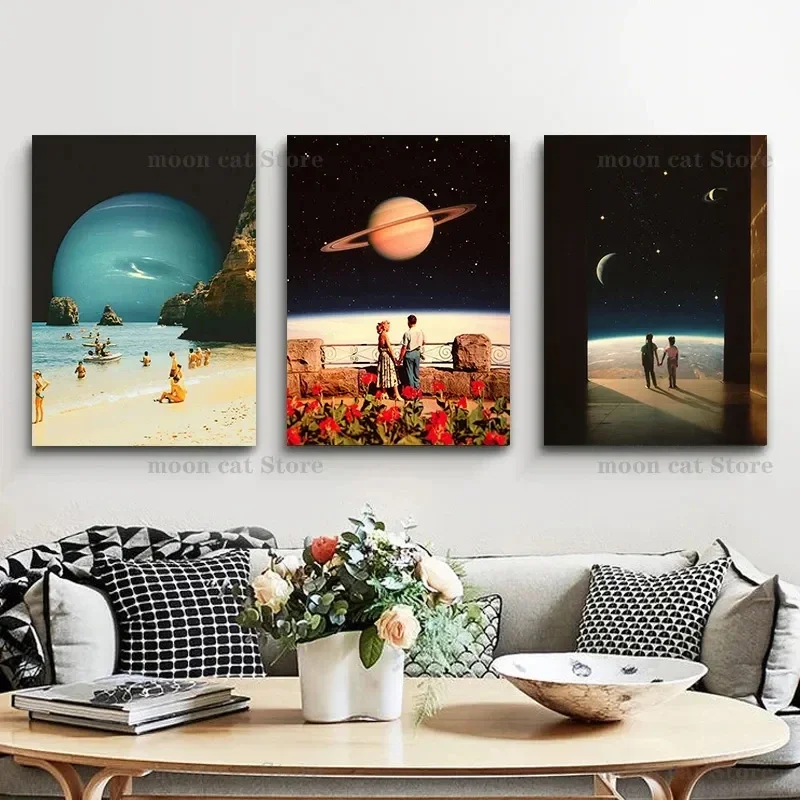The image appears to be a promotional photograph showcasing a stylish living room with contemporary decor. Dominating the scene is a grey couch adorned with black and white geometric pillows. Situated in front of the couch is a tan-colored coffee table topped with a vase of roses, a couple of coffee table books, and a decorative bowl. The wall behind the couch, painted light blue, features three striking sci-fi art prints. The left print depicts people on a beach by the sea with a massive globe on the horizon set against a black sky. The middle print showcases a couple holding hands on a balcony, gazing across clouds towards what appears to be Jupiter. The right print illustrates another couple holding hands, looking out over a distant planet in a cosmic setting. A subtle watermark reading "Moon Cat Store" suggests these prints are available for purchase. The overall scene blends modern home decor with captivating, space-themed artwork, creating an inviting yet otherworldly atmosphere.